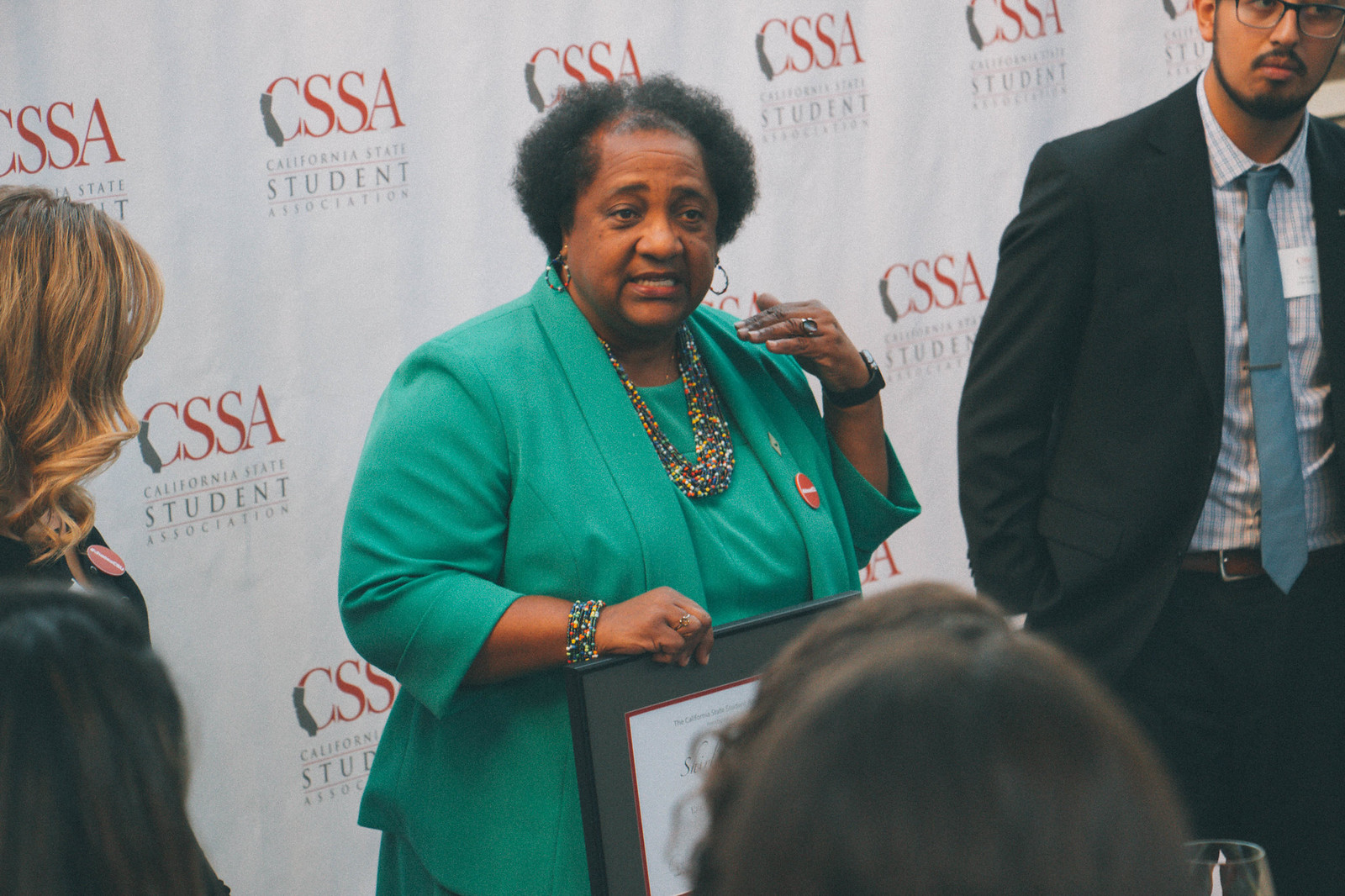The image captures a lively moment at the California State Student Association (CSSA) event, featuring an African-American woman, the central figure, who is engaging with the audience. She stands confidently, adorned with short, curly dark hair, gold hoop earrings, and a multi-layered array of colorful bead necklaces, complemented by a matching bracelet. Her attire is a vibrant green suit, and in her hand, she holds a black-framed object, presumably a plaque intended for a student, though it is partially obscured by someone's head in the foreground. On her lapel, she sports a pin that is a red circle with a white line through the center.

To her left, the side profile of a woman with curled red hair and a black suit is visible. This woman also wears a similar pin on her lapel. On the right, a bearded man with glasses, dressed in a dark suit and blue tie, stands attentively. 

Behind them, the background features a prominently displayed white banner, repetitively emblazoned with the red CSSA logo and the full name "California State Student Association" every six inches, framing the distinguished gathering with a uniform and professional touch. The gentleman in a sports coat, tie, and suit, mentioned initially, seems to be the bearded man beside the central figure.